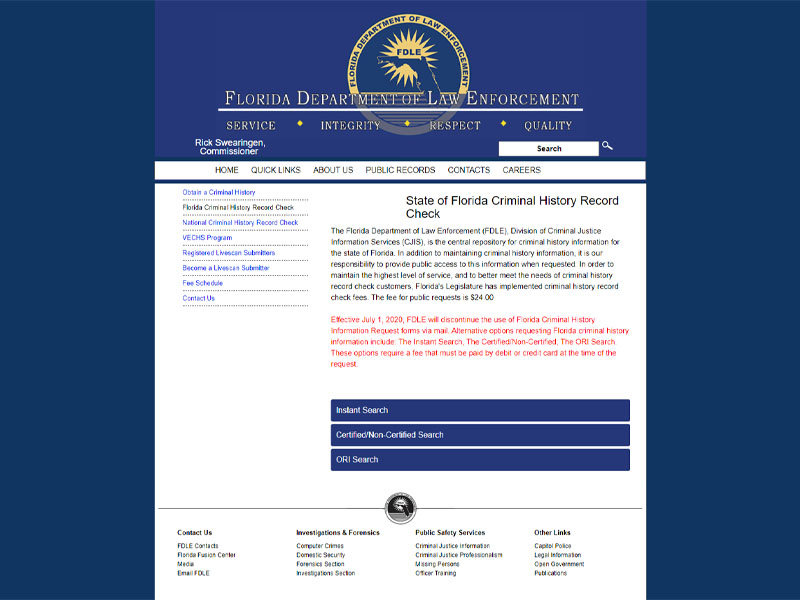The Florida Department of Law Enforcement (FDLE) is dedicated to service, integrity, respect, and quality, under the leadership of Commissioner Rick Schweringen. The FDLE acts as the central repository for criminal history information for the State of Florida. This responsibility includes maintaining and providing public access to criminal history information upon request.

On July 5, 2020, FDLE implemented a fee schedule for obtaining a Florida criminal history record check, set at $24.00 per request. This fee aims to better meet the needs of those seeking criminal history record checks. The service includes both certified and non-certified searches.

Additionally, the FDLE operates within the Division of Criminal Justice Information Services to manage and disseminate this crucial information efficiently and effectively. Public reference and contact avenues are established for individuals requiring a criminal history record check, whether for Florida-specific records or national criminal history checks.

To further streamline this process, Florida’s registrar has submitted protocols for criminal history record checks, ensuring timely and accurate information for the public's needs. This comprehensive system highlights FDLE’s commitment to upholding justice and maintaining the highest standards of service.